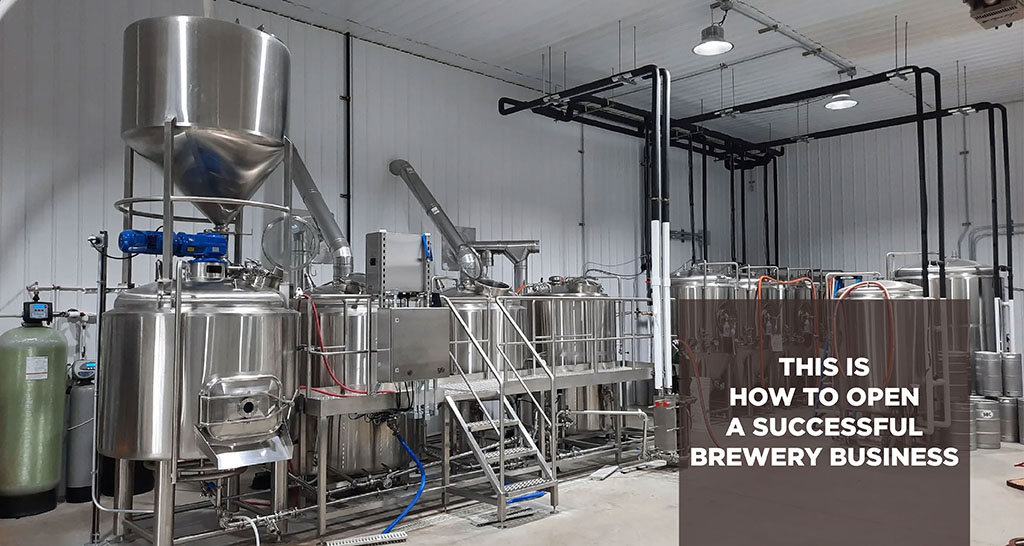This detailed image captures the interior of a brewery, showcasing a meticulously arranged assembly of shiny stainless steel brewing equipment in a well-lit, indoor setting. Dominating the corner of the room, a large cylindrical vat with a spout transitions into another vat via a tapered bottom. Interposed between these vats is a blue cylindrical element, likely serving as a filtration unit. Adjacent to this setup, a small mezzanine, accessed by a short ladder or stairway, allows operators to manage three additional cylindrical vats—two of which are fitted with wall-attached exhaust pipes.

To the left of the initial vat are two additional cylinders, one green and the other gray, each equipped with monitors displaying vital readings. Extending from the mezzanine structure, a network of black and white pipes snakes upward from the floor to the ceiling, running towards the corner and interconnecting with more vats aligned along the back wall. This back wall, characterized by its white, corrugated iron surface, is partially obscured by yet another series of vats. The bottom right-hand corner of the scene features a cluster of kegs neatly arranged.

The industrial environment is well illuminated by overhead lights suspended from the ceiling, casting a clean, well-maintained look across the space. A light brown box in the bottom right-hand corner of the image displays the text, "THIS IS HOW TO OPEN A SUCCESSFUL BREWERY BUSINESS," written in bold, white uppercase letters.